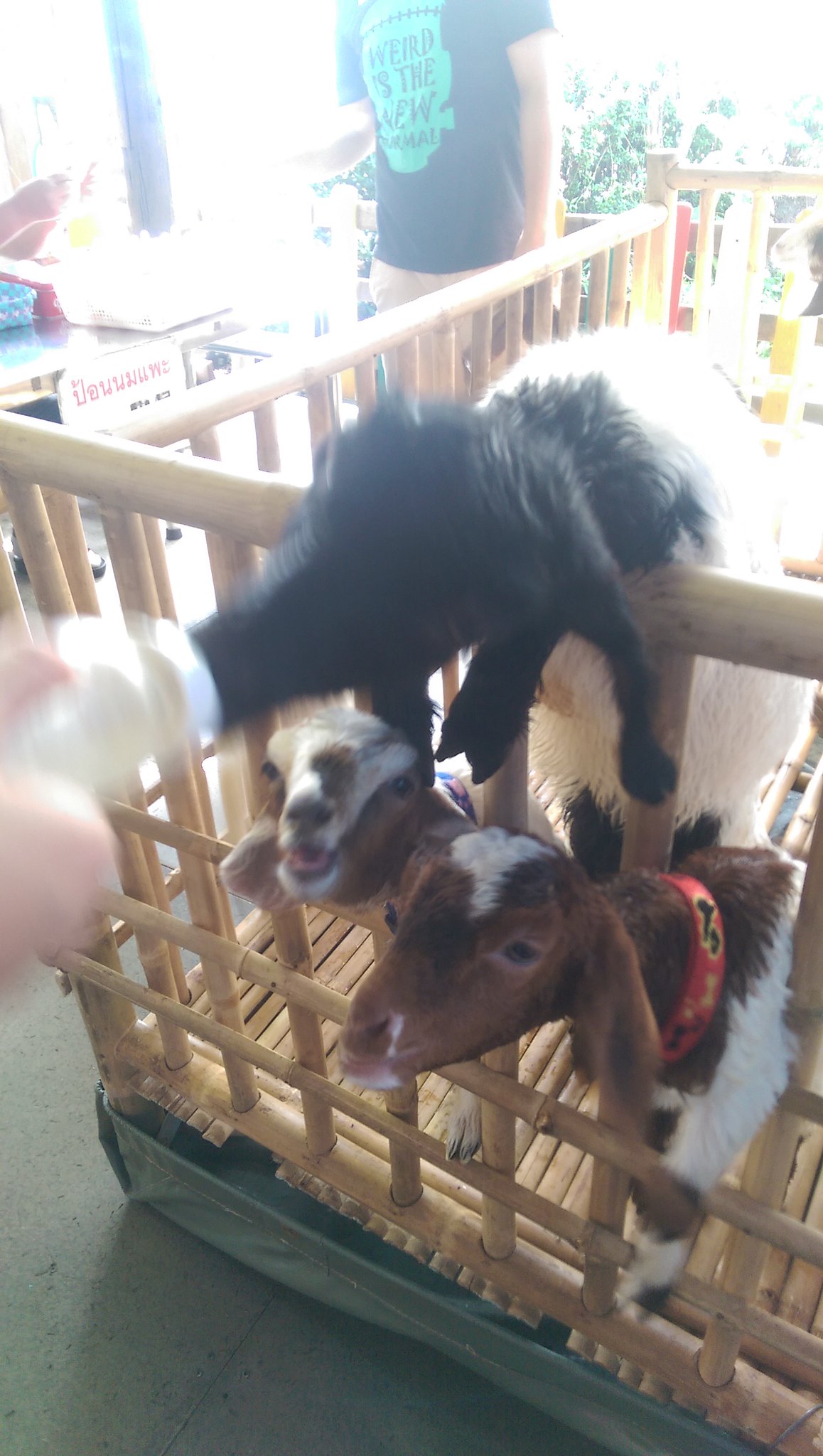The photograph captures a wooden pen reminiscent of a large crib, constructed from bamboo-like sections of wood. Inside the pen, three goats are featured: two young ones with brown-and-white fur, one with a distinctive red collar and a white leg. These two are more prominently on the ground, and one has its mouth open eagerly. Perched atop the pen's fencing is a larger, possibly adolescent goat, partially blurred in the image, with only its neck and paws clearly over the fence. The scene includes a human hand, also somewhat blurred, holding a bottle, suggesting the goats are being fed. The overall image is brightly lit, capturing the lively nature of the setting, which appears to be an event where people gather to view and interact with the animals. In the background, hints of writing and a person in blue clothing indicate an organized display or petting area, with some blurred areas adding a dynamic feel to the scene.